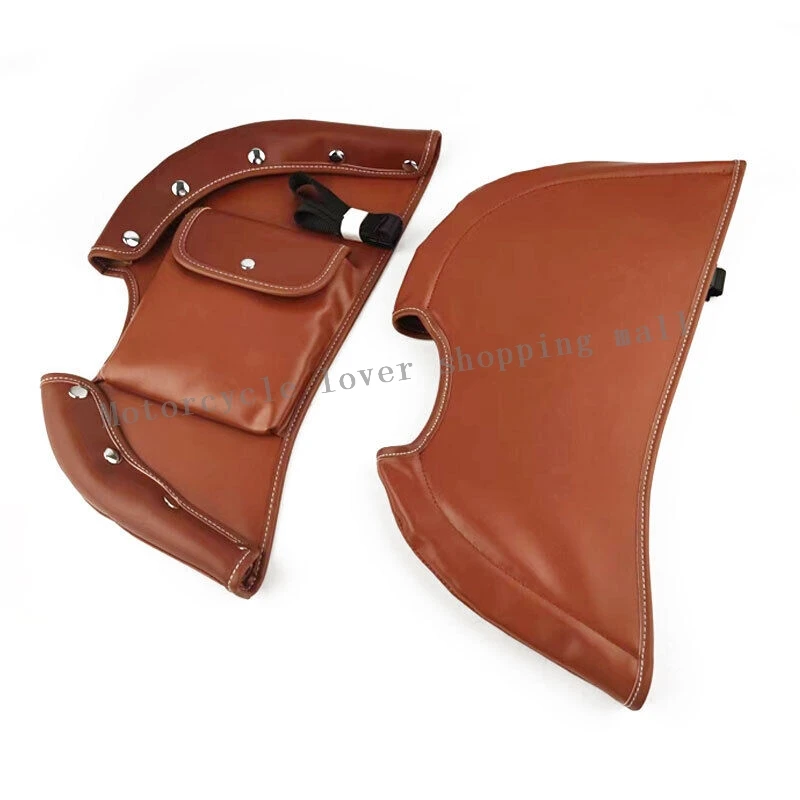The image features a brown leather pouch displayed on a white background, showcasing both sides of the item. In the center, there is a smaller, semi-circular coin purse-like pocket with a metal clasp, complemented by silver rivets along the folded edge. The left side reveals these rivets as well as additional detailing such as a shoelace-like lace above the pocket. The right side is smooth leather, marked with yellow stitching. Superimposed diagonally over the pouch in gray text, "Motorcycle Lover Shopping Mall" serves as a watermark. The overall shape of the pouch is reminiscent of half a pizza or dome, suggesting that it might be a two-piece accessory designed to attach to a motorcycle.